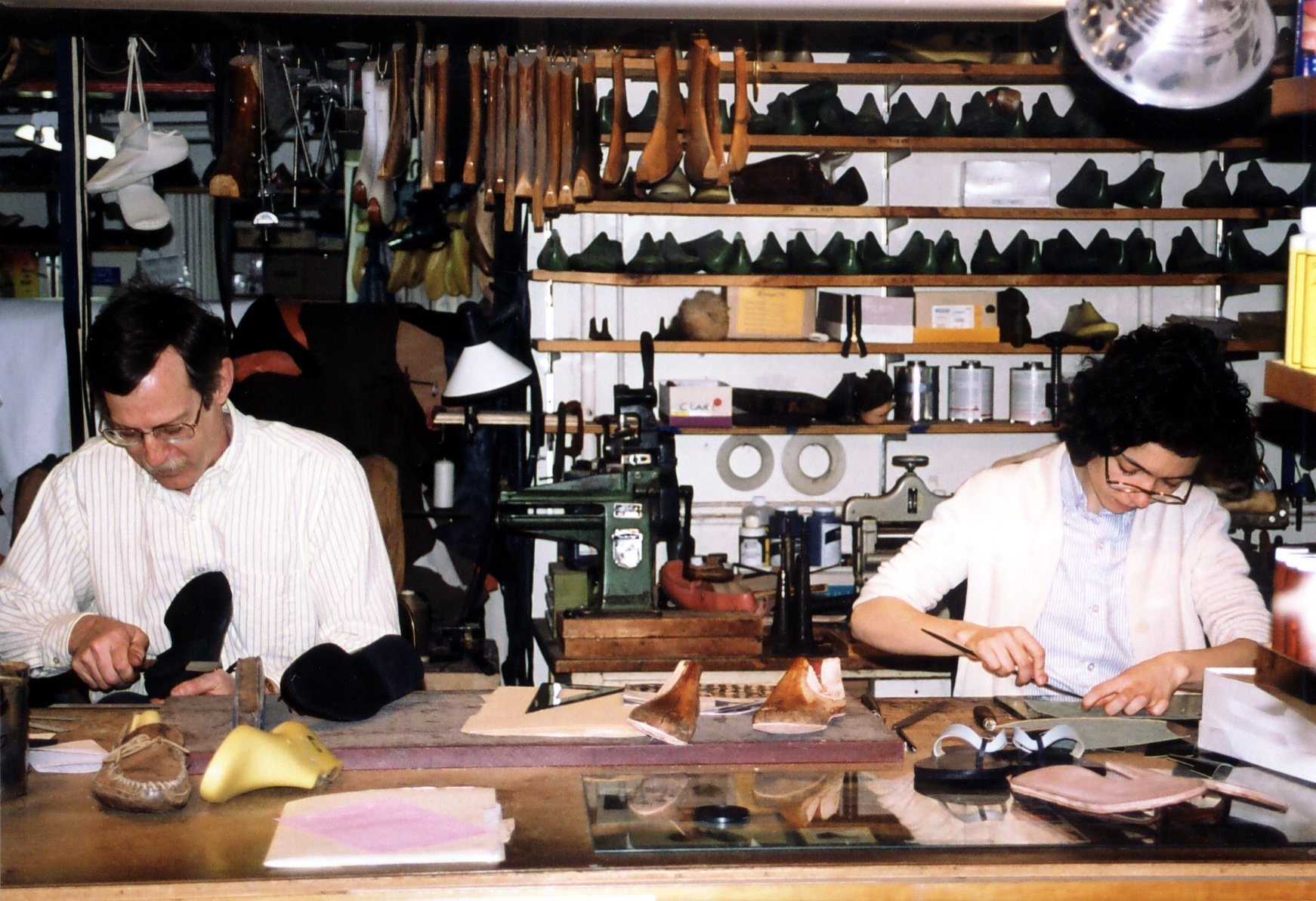This photograph captures a busy, vintage-style cobbler's workshop with two individuals intensely focused on their shoemaking craft. Seated at a large wooden workbench, the man is positioned on the left, identifiable by his dark hair, glasses, and grey mustache. He wears a white pinstripe shirt and is engrossed in working on the sole of a black shoe, holding a nail and possibly using other hand tools. To his right, a woman with dark curly hair and glasses, which rest halfway down her nose, is also deeply engaged with her work, wielding a long, pointed tool. Scattered across the table are various cobbler tools, wooden shoe molds, pieces of sandals, shoe soles, and a variety of footwear, including a brown moccasin and a pale yellow boot.

The backdrop is densely packed with shelves holding an array of shoes and cobbling equipment. Overhead, gooseneck lamps illuminate the workspace, and the shelves display a mix of leather shoes and boots, with notable items like a pair of hanging white sneakers or moccasins. The wall also features hanging leather pieces and numerous cobbler tools, further emphasizing the workshop's purpose.

The image, likely an old photograph taken with a camera rather than a modern phone, exudes a nostalgic, retro vibe, reminiscent of days when shoemaking by hand was more common. The scene is rich with details, suggesting a snapshot from a time when craftsmanship prevailed, making it a fascinating glimpse into the world of traditional shoemaking.